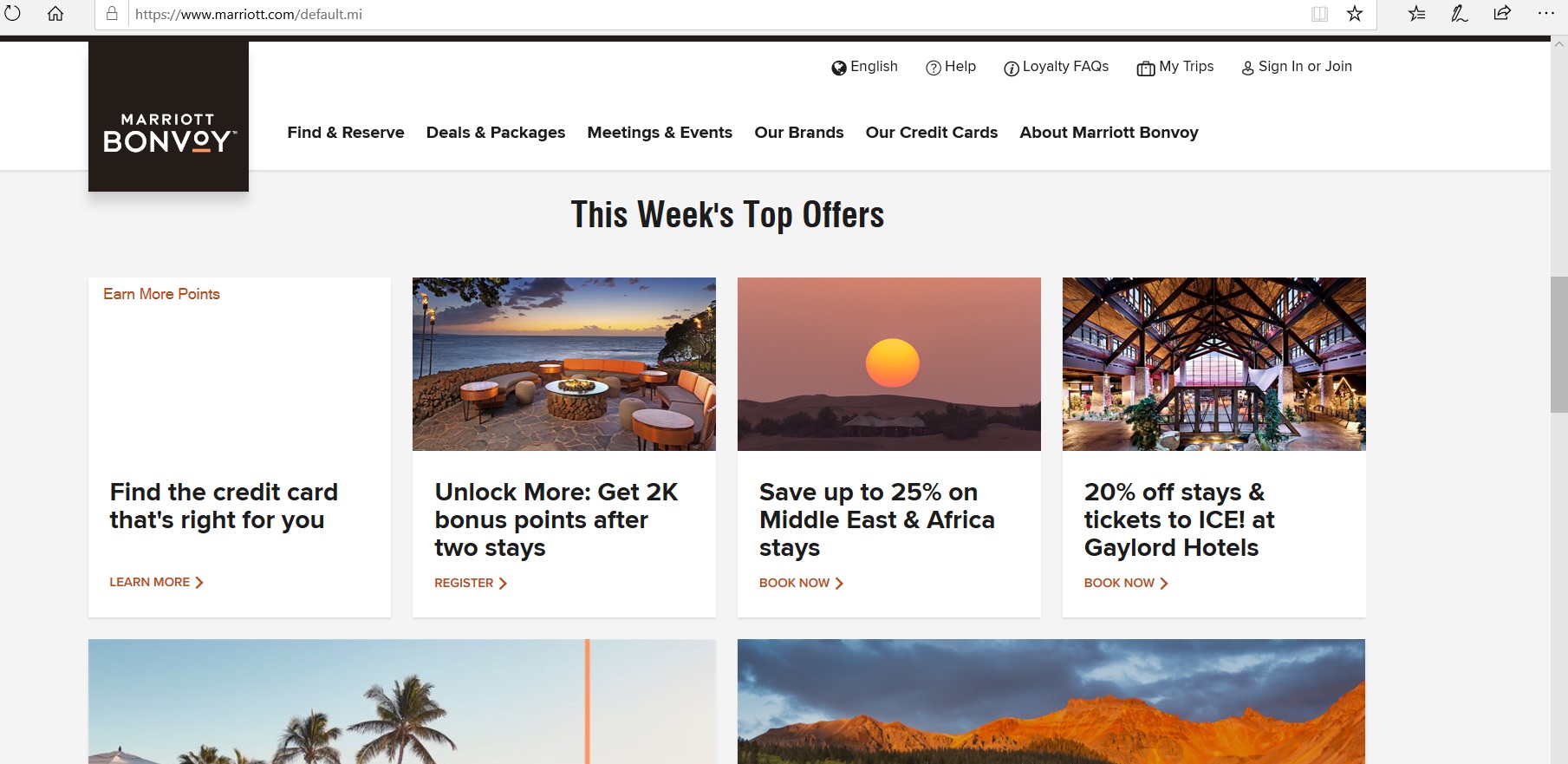The image depicts the Marriott Bonvoy website interface. At the very top, a URL bar is visible, indicating the website link. The page background features a light gray color on both the left and right sides. Directly beneath the URL bar are several navigation categories: "Final Reserve," "Deals and Packages," "Meetings and Events," "Our Brands," "Our Credit Cards," and "About Marriott Bonvoy."

Just below these categories, the section titled "This Week's Top Offers" is displayed. This section includes four white square icons, each representing a different promotional offer. The first icon is about finding the right credit card, the second highlights a promotion for unlocking a bonus of 2,000 points after two stays, the third offers savings of up to 25% on stays in the Middle East and Africa, and the fourth advertises a 20% discount on stays and tickets to ICE at Gaylord Hotels.

Further down, the page features an image of palm trees set against a light blue sky. Adjacent to this image, on the right side, is a depiction of an orange rocky mountain under a similarly blue sky. A scroll bar is located in the center-right of the page, rounding out the visual elements from top to bottom.